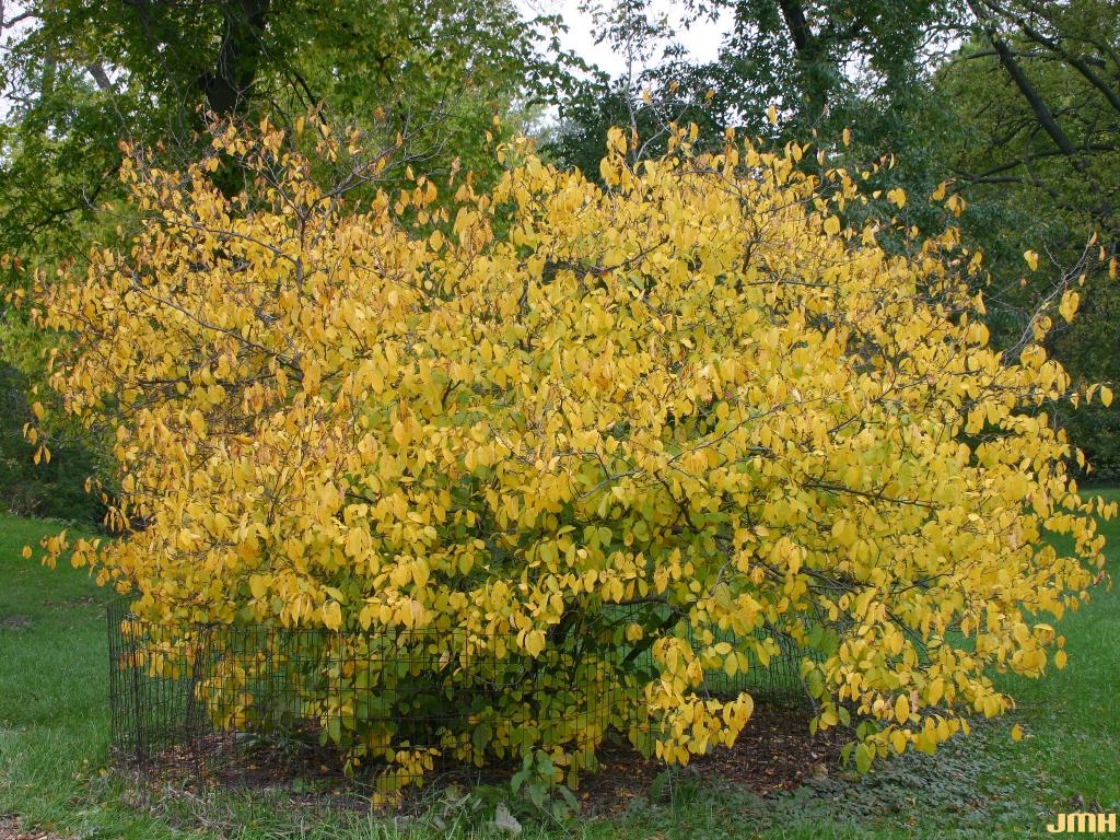In the center of the image is a broad, low bush with vibrant yellow leaves, standing out prominently against the scene. The bush is surrounded by a chicken wire fence, and its base rests on a brown dirt floor, edged by a grassy area. The leaves vary in shade, with a mix of bright yellow, darker yellow, and a few brown and light green leaves. Some stems are visible through the dense foliage, and a few branches extend outward. Behind the bush, the landscape transitions into a dense forest of tall trees with green leaves, their trunks forming a textured backdrop. Patches of blue sky seep through the tree canopy, adding depth to the scenery. The bottom right corner of the image is marked with the yellow block initials "JMH," possibly the artist's signature.